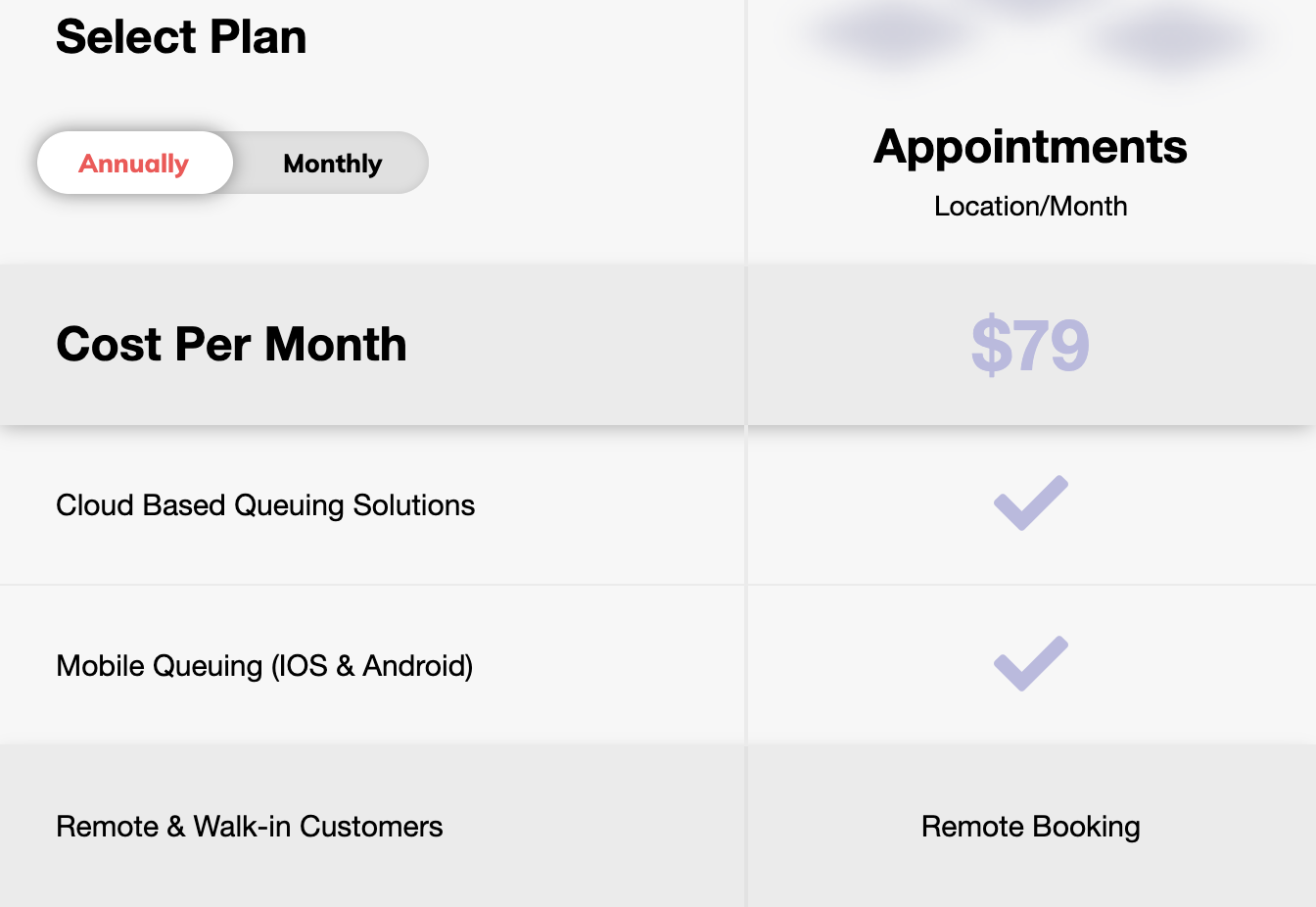**Image Description: Plan Selection Chart**

The image features a detailed plan selection chart for a service, allowing users to choose between annual and monthly payment options. 

**Left Column:**
- **Header:** "Select Plan" (bold, black box)
- **Payment Options:**
  - *Annual* (red font, currently selected)
  - *Monthly* (standard font)
- **Plan Details:**
  - **Cost per Month:** 
    - Cloud-Based Queuing Solutions
    - Mobile Queuing (iOS, Android)
    - Remote and Walk-In Customers

**Right Column:**
- **Feature Availability:**
  - **Cost per Month:** $79 (light purple font)
  - **Cloud-Based Queuing Solutions:** Checkmark (indicating availability)
  - **Mobile Queuing:** Checkmark (indicating availability)
  - **Remote and Walk-In Customers:** Listed as "Remote Booking"

The chart provides a clear comparison of features, with the selected payment plan (annual in this case) highlighted in red to show its active status.